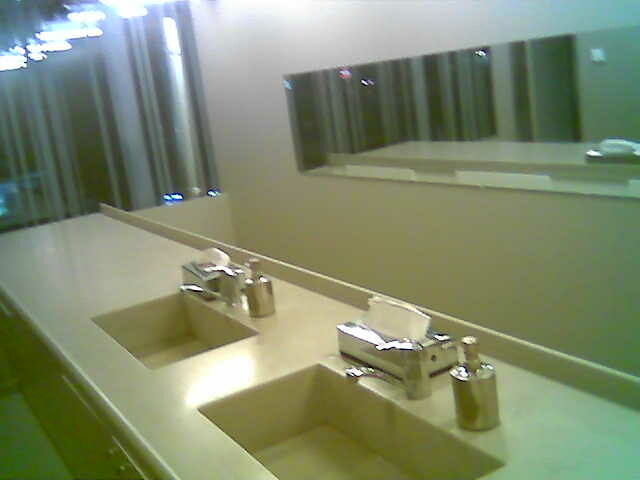This photograph captures the interior of what appears to be a public restroom. The focal point is a long, unframed mirror that spans the back wall from the bottom right to the upper left, reflecting the meticulous setup of the wash area. In front of this mirror sits a double vanity with two deep, rectangular sinks positioned centrally on the counter. Each sink is equipped with a sleek, silver faucet. To the right of each faucet, there is a silver soap dispenser, while to the upper left, a silver Kleenex box with tissues protruding adds a touch of practicality. The left side of the image hints at large windows or mirrors with vertical silver lines, possibly blinds, contributing to the illumination provided by ample overhead lighting. The setting gives an impression of an expansive, well-lit bathroom with a clean and modern aesthetic. The reflection in the mirror replicates this organized scene, enhancing the sense of spaciousness by showing more of the counter and the fixtures.